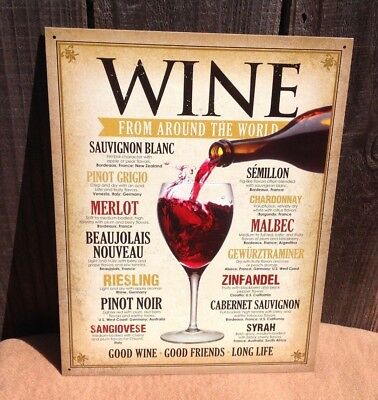This is a color photograph of a tan artistic sign, propped up on a light brown tabletop surface in front of a dark brown, weathered wooden fence or wall. The sign has an ornate border and prominently reads "Wine From Around the World" at the top, with a yellow ribbon surrounding the text. Central to the image is an amber-brown wine bottle positioned from the right-hand side, pouring dynamic streams of red wine into a nearly full wine glass, causing a slight splash. Flanking the wine glass, listings of various wine names stretch from top to bottom on both the left and right sides. On the left, the wines are: Sauvignon Blanc, Pinot Grigio, Merlot, Beaujolais Nouveau, Riesling, Pinot Noir, and Sangiovese. On the right, the wines listed are: Semillon, Chardonnay, Malbec, Gewürztraminer, Zinfandel, Cabernet Sauvignon, and Syrah. Underneath each wine name, there are small, unreadable descriptions. At the bottom of the sign, it reads "Good Wine, Good Friends, Long Life."